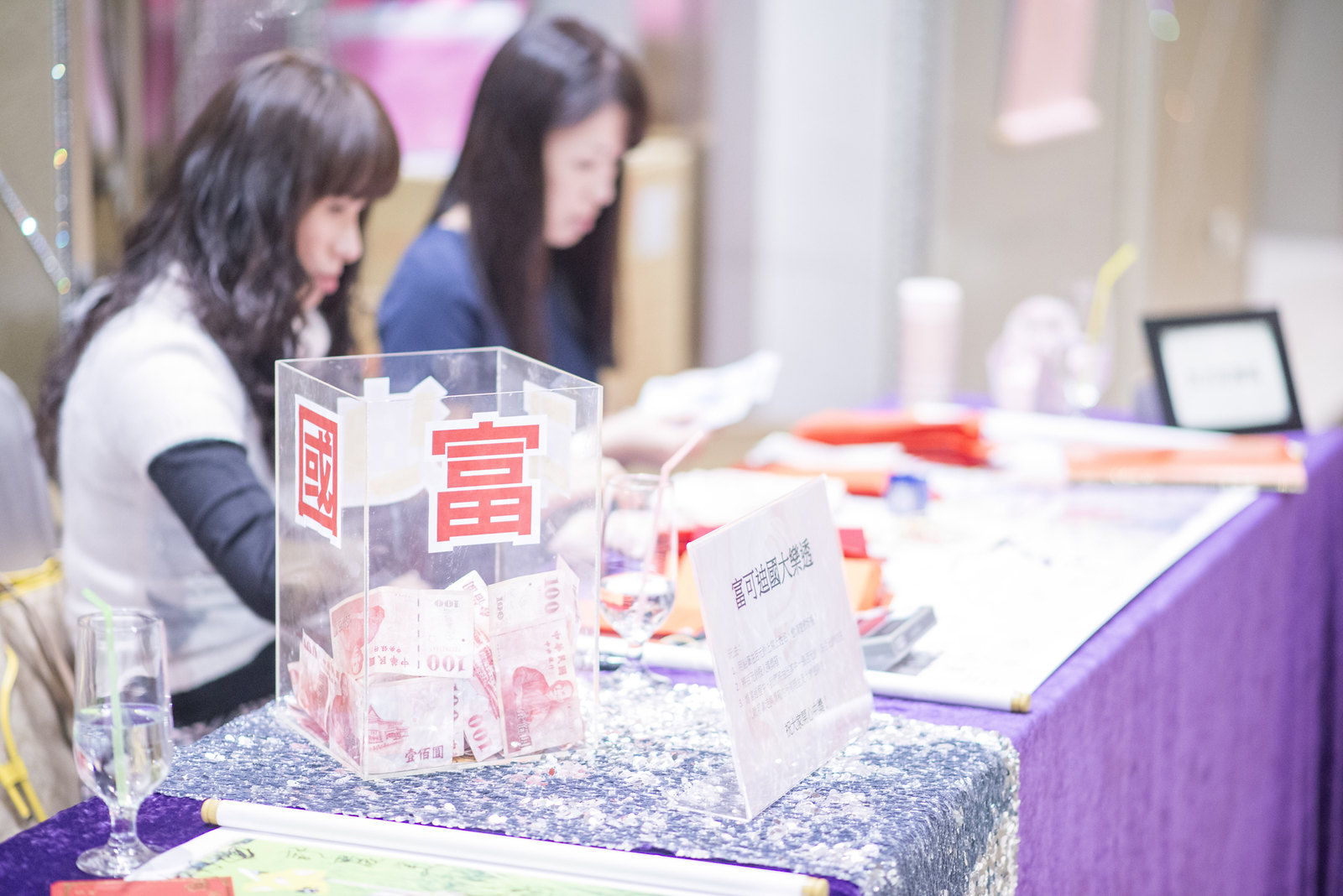In this photograph, two women of Asian descent are seated at a long rectangular table adorned with a purple tablecloth. Both have long, dark hair—the woman on the left wears a grey shirt with black sleeves, while the woman to her right also has black hair. The image is taken at an angle, causing parts of it to be slightly out of focus, particularly the women and the far end of the table. 

In front of them sits a variety of items, most notably a large, clear acrylic box containing foreign currency, distinguishable by its white background and red text, along with characters in another language, likely Chinese. There's a paper sign in front of the box, though its contents are unreadable. Also visible in the bottom left corner is a stemmed drinking glass filled halfway with clear liquid, featuring a green plastic bendable straw. 

The setting suggests an environment where the women might be engaged in an activity or service that involves receiving tips, evidenced by the cash-filled box. Overall, the scene is rich in detail and hints at a functional setup possibly related to an event or market.